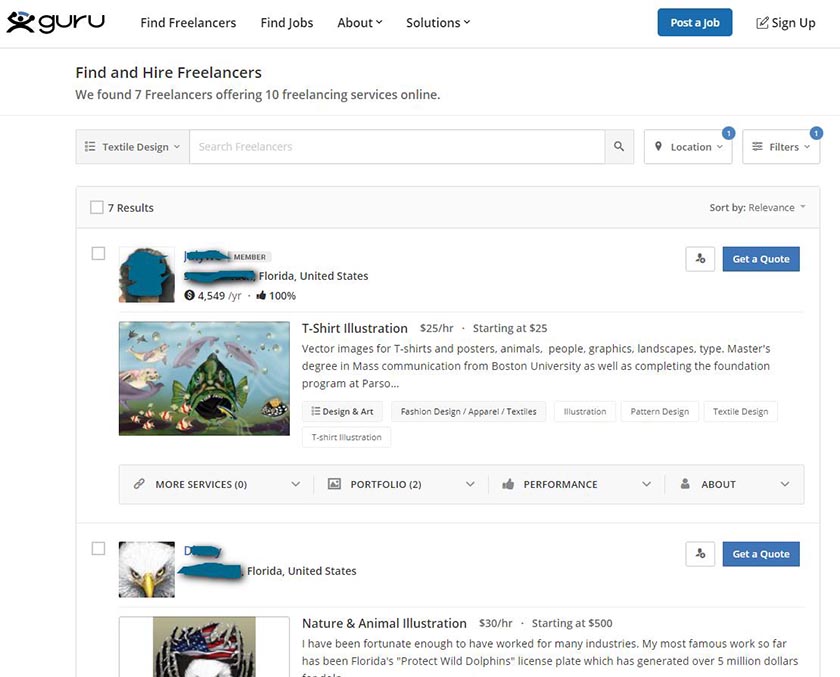**Detailed Caption:**

In this image, we observe a comprehensive view of an online freelancing platform's interface. 

- **Top Left Section:** At the top left corner, prominently displayed in black text, is the word "Guru." Adjacent to it on the left, the platform's logo features a human figure holding a blue, rainbow-like arc above their head.
  
- **Navigation Menu:** To the right of the "Guru" text, there is a horizontal navigation menu comprising several categories:
  - "Find Freelancers"
  - "Find Jobs"
  - "About" (accompanied by a downward-pointing arrow, indicating a dropdown menu)
  - "Solutions" (also accompanied by a similar downward-pointing arrow)

- **Top Right Section:** 
  - The "Sign Up" button is situated at the top right corner, identifiable by an icon depicting a paper and pencil.
  - To the left of the "Sign Up" button is another button labeled "Post a Job."

- **Central Top Section:**
  - On the left side of this section, a heading reads "Find and Hire Freelancers."
  - Beneath this heading, an informational text states, "We have found 7 freelancers offering 10 freelancing services online."

- **Search and Filter Options:**
  - Below the informational text, within a framed box, is the label "Textile Design."
  - Adjacent to this boxed label, another text box provides an input field labeled "Search Freelancers."
  - Farther to the right are two additional filter options:
    - A box labeled "Location," marked with a "1" at the top right corner.
    - To its immediate right, another box labeled "Filters," also marked with a "1."

- **Freelancer Listings:**
  - Directly below the filtering options, two freelancer services are prominently displayed:
    - "T-Shirt Illustration"
    - "Nature and Animal Illustration," positioned at the bottom middle of the image.

This detailed layout showcases the navigational and functional elements of the freelancing platform's main page, highlighting key features for users to find and hire freelancers.